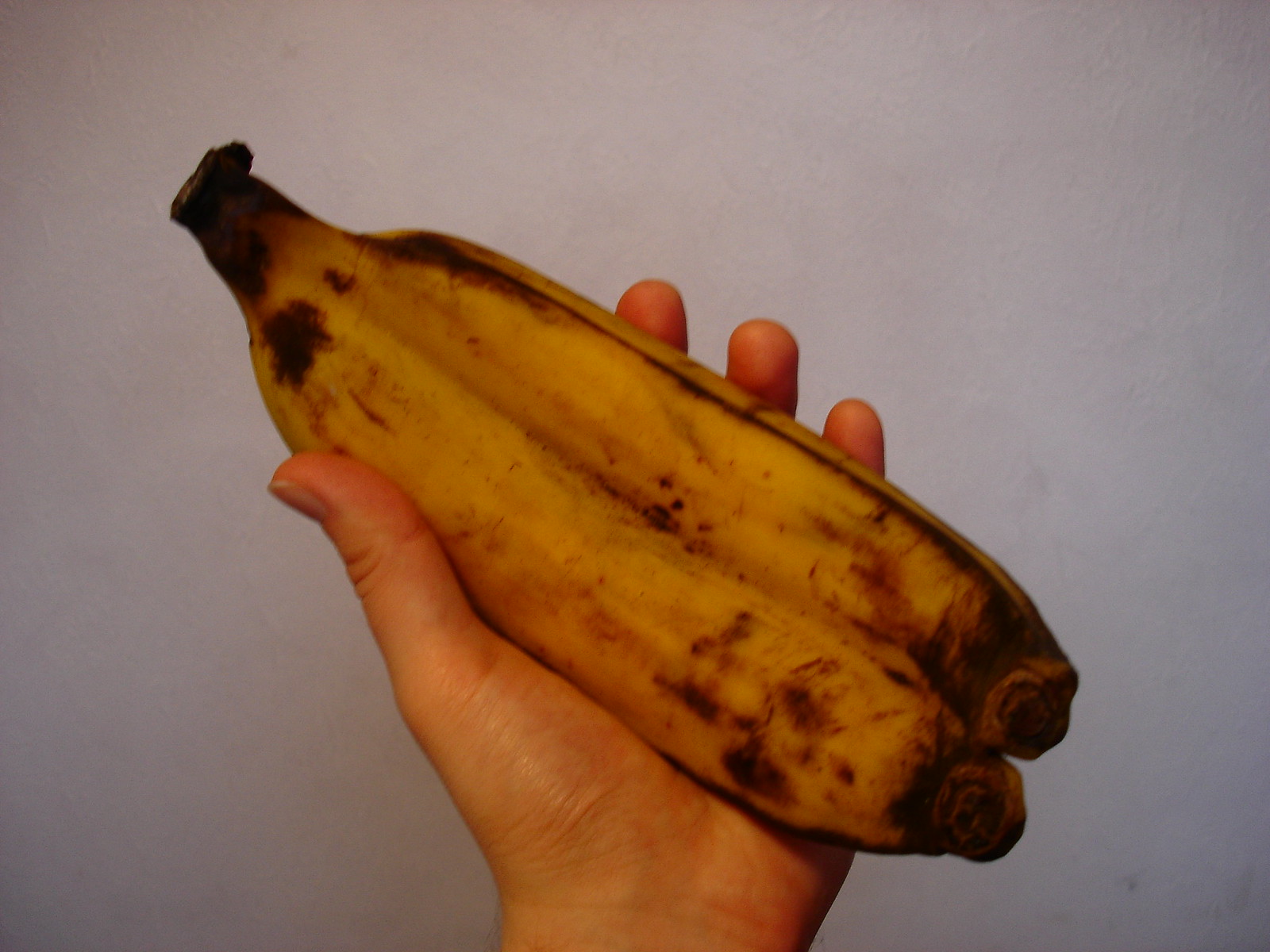The grainy photograph captures a left hand holding two attached bananas against a blank white wall. The hand, visible with the thumb wrapping around the front and three fingers supporting the back, holds the bananas that exhibit significant signs of overripeness. Various brown spots cover the sides, and the banana on the right features a prominent brown line. The banana on the left appears slightly larger than the one on the right. Despite the image's poor quality, the distinct details of the bananas' condition are clearly discernible.